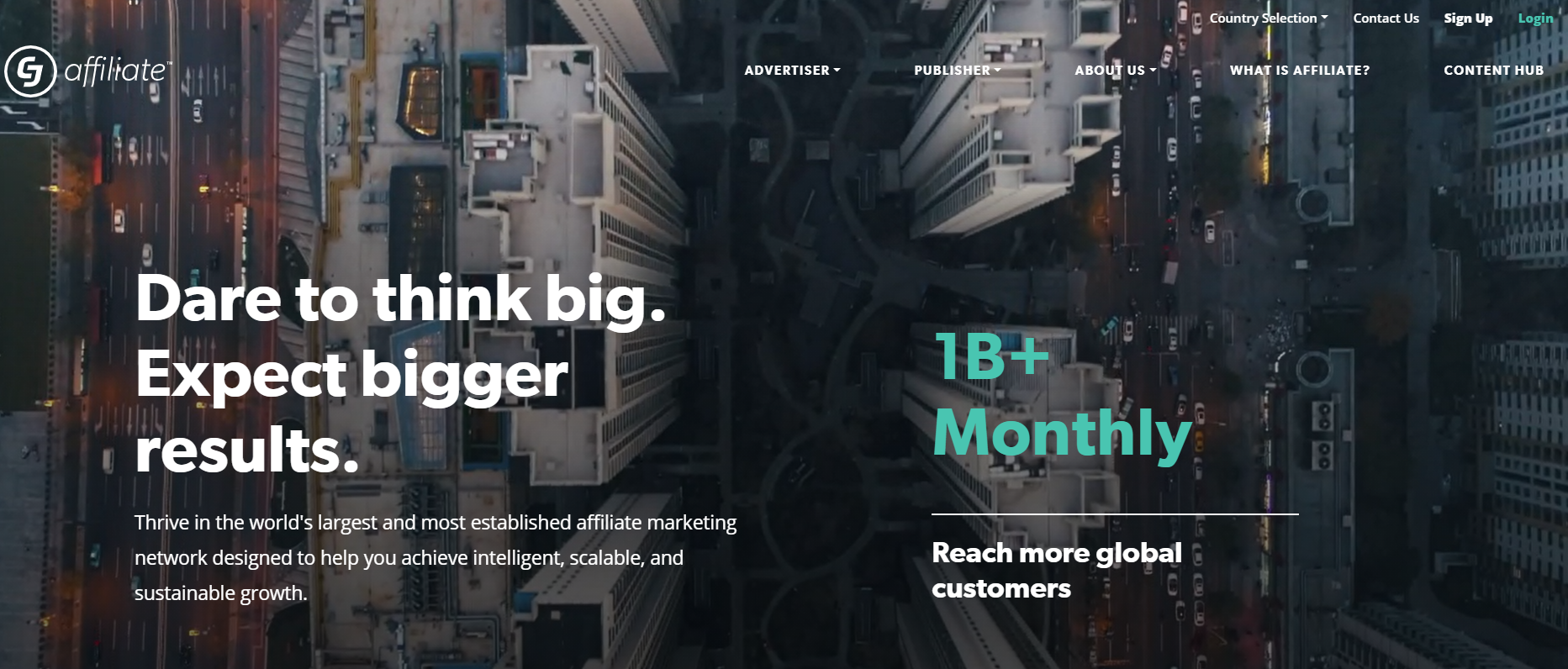Here's a cleaned-up and detailed caption:

---

"An aerial photograph of towering skyscrapers graces a bustling business website. The roofs of these high-rise buildings dominate the view, embodying the heights of ambition. Prominently displayed text encourages visitors to 'Dare to think big, expect bigger results,' followed by smaller, unreadable text. Below, a bold claim announces, '1 billion+ monthly, reach more global customers.' A logo, resembling either a 'G' or an 'S', is accompanied by the word 'affiliate', suggesting a connection to global outreach or marketing. On the right side of the webpage are several drop-down menus, though their detailed content remains unclear. Despite the powerfully inspiring message, the website lacks clear branding, making it difficult to identify the company behind it."

---

This caption provides a thorough and descriptive overview of the webpage, highlighting both its visual and textual elements.